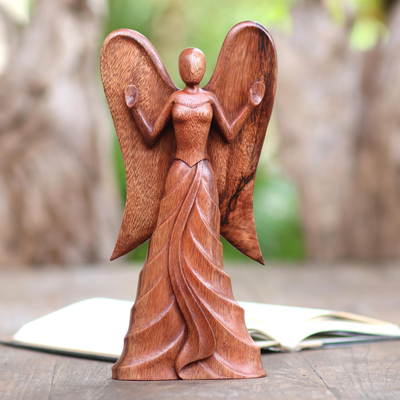In an outdoor setting bathed in daylight, set against a backdrop of blurred tree branches, leaves, and dappled sunlight, there is an intricate, small wooden sculpture positioned on a table-like surface. The sculpture, carved from wood with varying shades, portrays a female angelic figure with smooth, rounded wings that taper to sharp points. The angel’s arms are raised and connected to the wings, palms outward, blending into the natural contours of the wood. The figure lacks distinct facial features, showcasing only a bald head with a subtle nose protrusion. Adorned in a layered skirt that extends down to a point, the sculpture includes a front tie detail and a sash-like design that elegantly divides the skirt. The wood's natural grains are prominently visible, particularly a dark vein running through one of the wings, adding to its rustic charm. Placed just behind the sculpture is an open book with white pages, further emphasizing the scene’s serene and contemplative atmosphere. The predominant colors in the image are whites, blacks, various shades of green, and rich browns, enhancing the detailed craftsmanship and natural beauty of the composition.